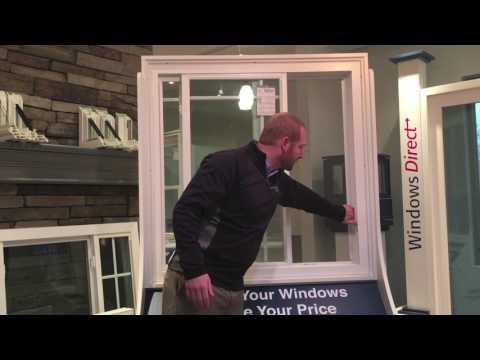In the color photograph, which is in landscape orientation, a man with short red hair and a beard stands at the center, slightly facing the right side. He is dressed in a black zip-up jacket and beige trousers. He appears to be demonstrating the functionality of a large window frame that is partially open and slightly crooked. His left hand is reaching out to touch the edge of this window frame. Positioned in the center of the frame, he looks down slightly at the windowsill behind him. To the right of him, there is another window frame.

A horizontal black strip runs across the top and bottom of the image, and text on the image reads, "Windows Direct, Your Windows, Your Price," with "Windows" in dark blue and "Direct" in red. This text is visible on a vertical post to the left of the main window, and beneath the window frame, part of the text reading “Your Windows at Your Price” is partially obscured by the man. 

In the bottom left corner of the image, another window panel is seen propped against a stone wall. The background colors and elements in the image predominantly feature shades of gray, white, black, red, and dark blue. The overall setting suggests a product showcase or a demonstration, potentially indicating a recent purchase or installation of the window.